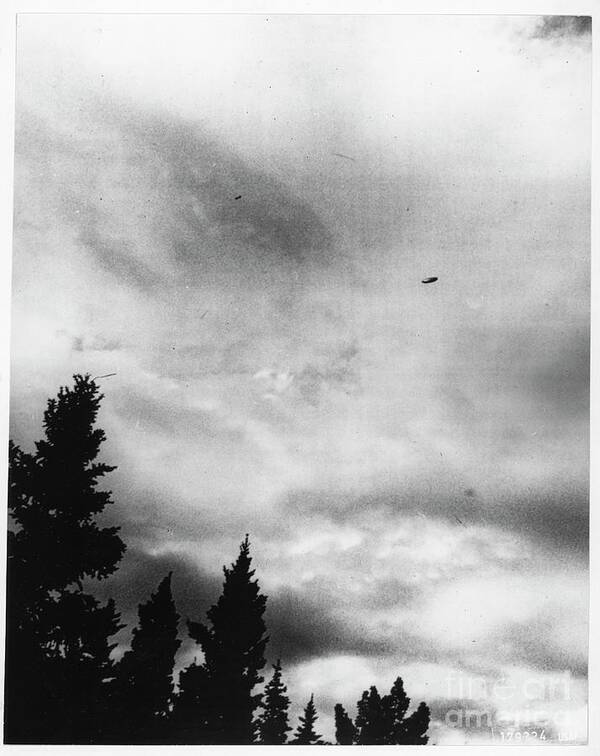This black-and-white photograph, captured by Fine Art America (Watermark visible in the bottom right corner), depicts an outdoor scene dominated by dense, ominous clouds filling the sky. The image is taken at an upward angle from the ground, featuring the tops of dark, evergreen trees clustered primarily in the bottom left-hand corner. The sky is mostly filled with gray clouds, contributing to a moody, almost dusk-like atmosphere. Amidst the clouds in the upper right portion of the image, about two-thirds of the way up, a small, saucer-shaped object can be discerned, resembling a UFO or possibly a plane, adding an element of intrigue. The photographic style enhances the dramatic contrast and details, evoking a mysterious, almost otherworldly scene.